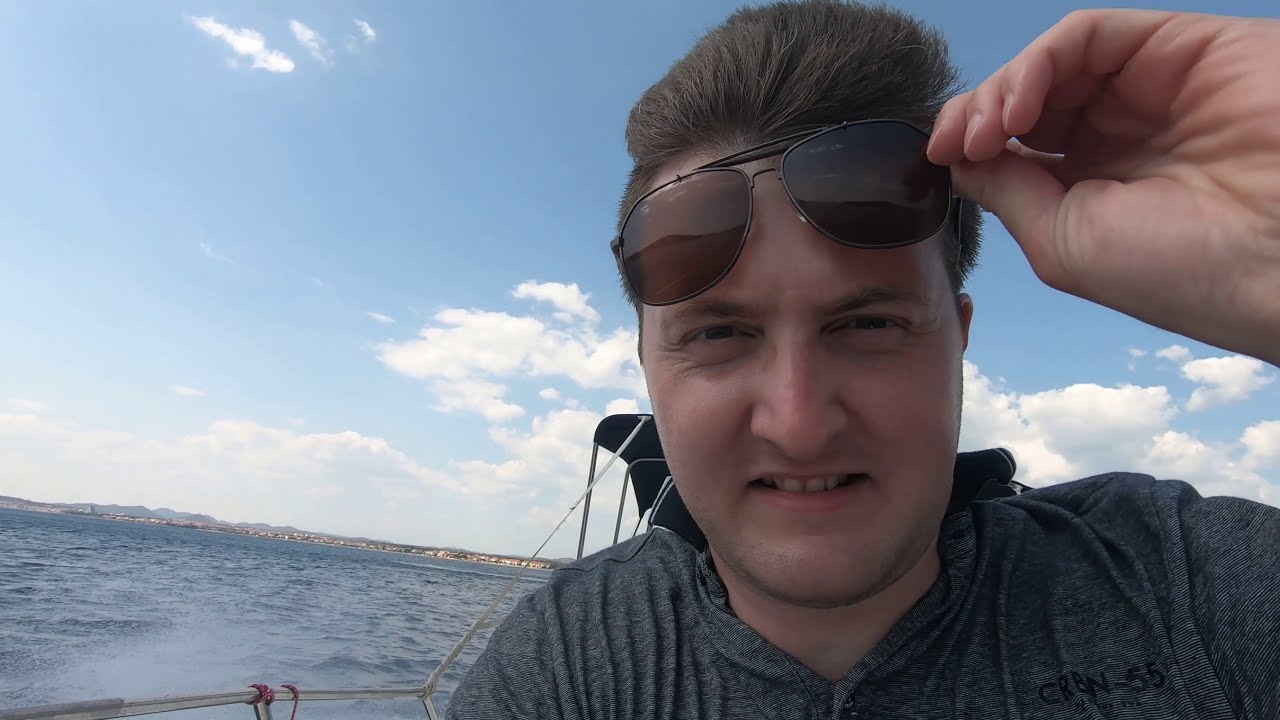A close-up of a man on a boat with a beautiful, sunny backdrop of a blue sky and puffy white clouds. The blue water with tiny ripples can be seen on the left side of the image, adding to the serene setting. The man, with short, light brown hair that sticks up due to the wind, is lifting large, round aviator sunglasses with a light brown tint onto his forehead using his right hand. His eyes are crinkled, showing crow’s feet as he squints and stares ahead, his mouth slightly open. He wears a light gray or heather gray lightweight jacket or long-sleeved shirt with 'CRBN-55' printed in black letters on the chest. The scene captures him as he takes a selfie, with the wind whipping through his hair, creating a dynamic and lively atmosphere.